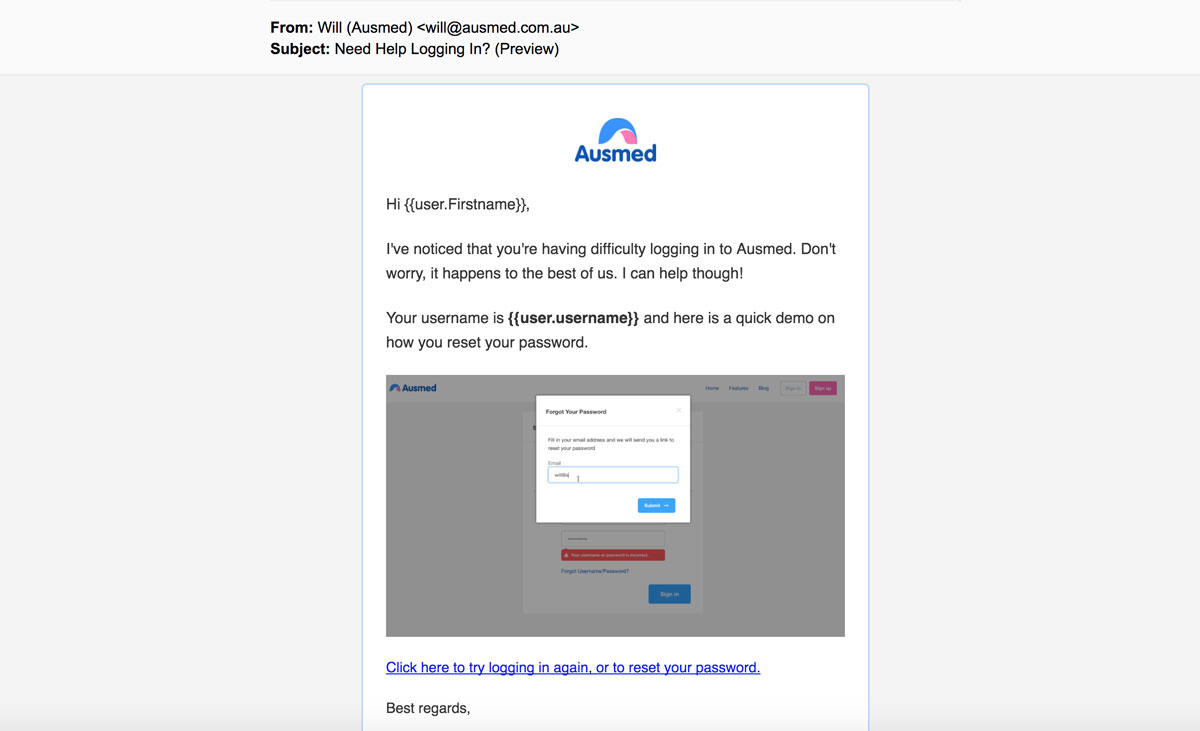A detailed caption for the image might read:

"This image features an email sent from Will Osmed of the company Osmed, with the sender's address as will.osmed.com.au, indicating that the company is based in Australia. The email's subject line, 'Need Help Logging In?' along with the sender's name, are both bolded. The email content is enclosed within a blue-outlined border. At the top center of the page, the Osmed logo, which is in blue and pink, is prominently displayed next to the bolded company name, 'Osmed.'

The body of the email starts with a greeting, 'Hi [user.first.name],' addressing the user personally. It acknowledges that the user is experiencing issues logging into Osmed: 'I've noticed that you're having difficulty logging into Osmed. Don't worry, it happens to the best of us. I can help though.' The email then provides the user's username, '[user.username],' in parentheses, and introduces a brief tutorial on resetting the password.

Below this introduction, there is a screenshot of the Osmed website. The image highlights the 'Forget Your Password' option and shows the process where the user needs to enter their email to receive a password reset link. A clickable link, highlighted in blue, is provided below the screenshot with the text, 'Click here to try logging in again or to reset your password.' The email concludes with 'Best regards.'

The overall design and layout signify a user-friendly and supportive tone from Osmed."